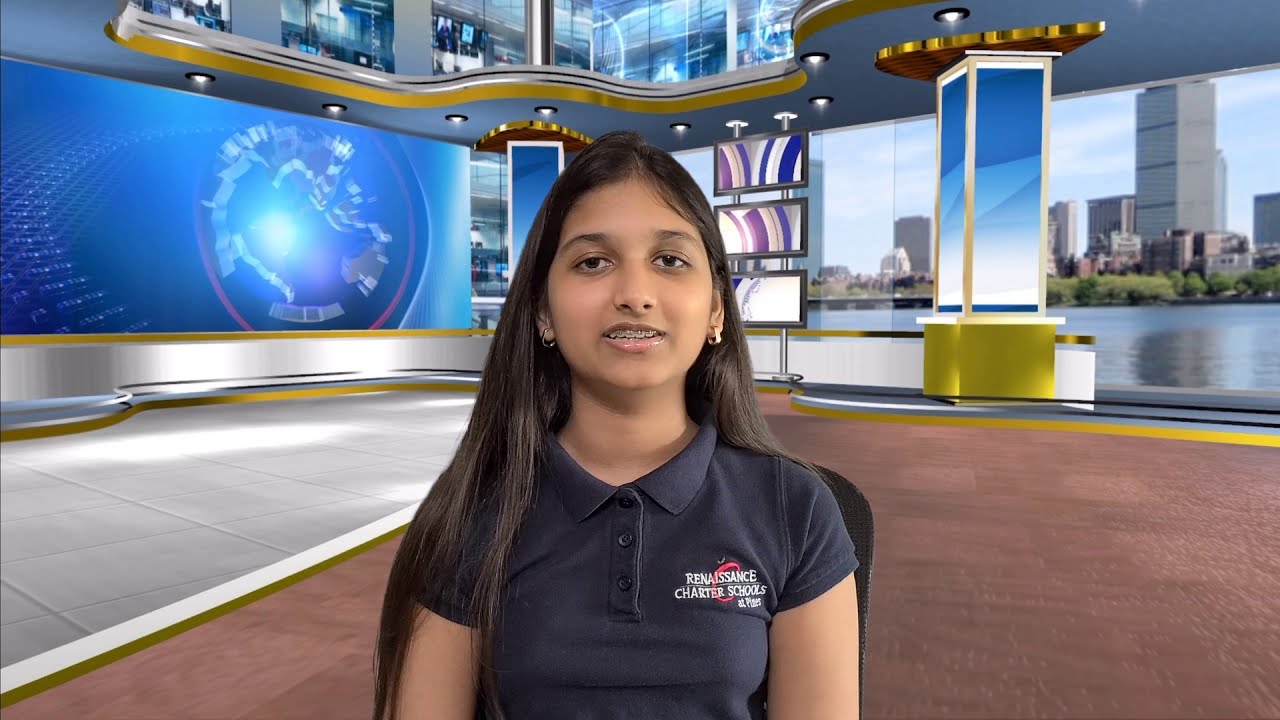This full-color indoor photograph features a young middle school girl with long, dark, brown hair and brown eyes, wearing earrings and braces, her mouth slightly open as she looks directly into the camera. She is dressed in a fully buttoned-up, navy blue polo shirt emblazoned with the name “Renaissance Charter Schools” alongside what appears to be a red apple logo. She sits in a chair against a highly detailed, colorful background that resembles a tech news studio, complete with blue lights, glass columns, and a cityscape. The background, likely a green screen, includes prominent sign boards and possibly a stylized image of the earth, giving the entire scene the sophisticated ambiance of a broadcast news setup.